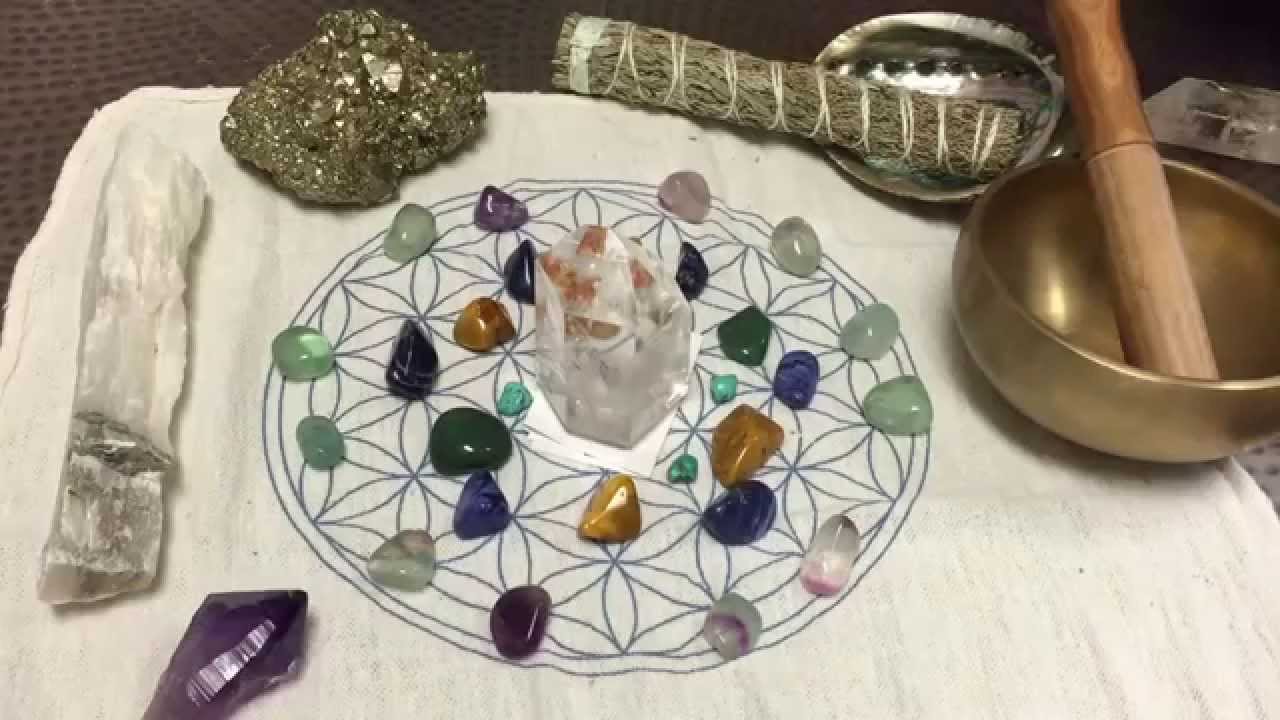This image captures an array of metaphysical supplies meticulously arranged on a white cloth draped over a table. The cloth features a complex, symmetrical design reminiscent of flowers within a hexagon, encircled by a larger circular pattern. At the center of this intricate design rests a large, transparent white crystal, around which a variety of differently colored stones, including rose quartz, malachite, and possibly moldavite, are strategically placed in a circular fashion.

In the lower left-hand corner, an elongated, pointed amethyst crystal stands out with its rich purple hue. Adjacent to this, a notable 10-inch long, clear white crystal extends vertically along the left side of the image. The top left corner showcases a dark gray pyrite stone, speckled with metallic flakes. Spanning across the top of the image lies a sizable bundle of sage, nestled in a shiny silver dish, adding a ritualistic touch. Meanwhile, the top right corner is adorned with a golden sound bowl, complete with a wooden implement, likely used for generating meditative sounds.

This well-balanced composition of crystals and metaphysical tools is not only visually striking but also evocative of a serene, spiritual ambiance.